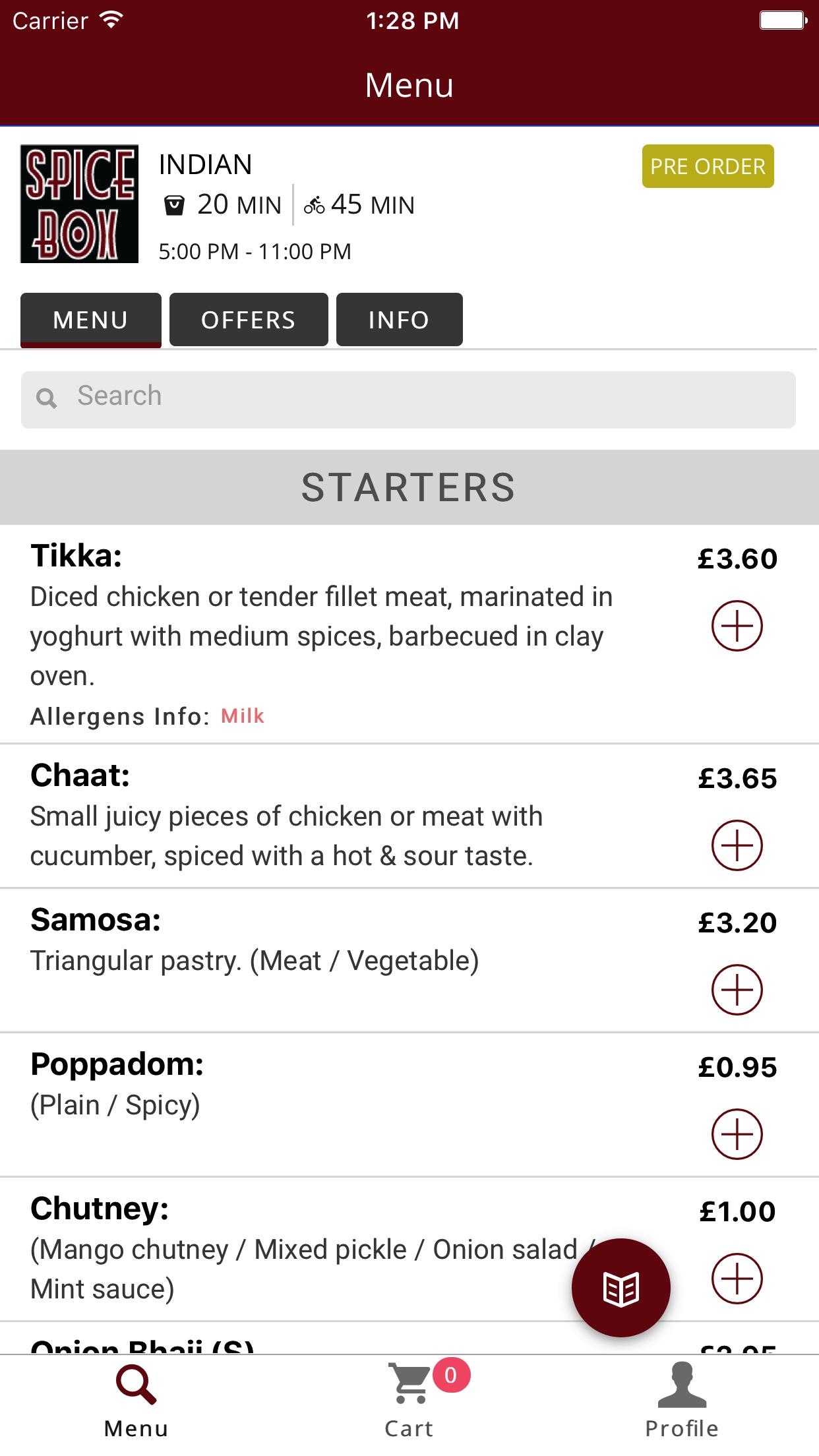Here is a more detailed and cleaned-up caption for the image described:

---

The image displayed is a screenshot of an Indian restaurant menu on a smartphone screen. At the top left corner of the screen, there is an indicator displaying the carrier information and the WiFi symbol. In the center top, the current time is shown as 1:28 PM. On the right side of the top bar, there is a full battery icon.

The interface contains a header with the restaurant name "Spice Boy," written in red text with a white border beside the restaurant's logo. Below the restaurant name, the word "Indian" is prominently displayed. There is an illustration of a take-out bag indicating a 20-minute preparation time for takeout orders, and a bike symbol suggesting a 45-minute delivery time. Next to these details, there is an option for pre-ordering in a gold text box, highlighting the available hours from 5 PM to 11 PM.

The main navigation options, "Menu," "Offers," "Info," and a search bar with a magnifying glass icon, are situated below the pre-order information. The search bar has a grey background.

The menu starts with a grey section labeled "Starters." The first item listed is "Tikka," offering diced chicken for €3.60 with a brief description underneath. Following this are "Samosa," priced at €3.20, and "Papadum" (noted as both plain and spicy), costing €0.95.

At the bottom of the screen, there is a row of icons including a book icon, which is currently selected, and other icons labeled "Menu," "Card," and "Profile."

---

This caption provides a clear, structured, and comprehensive description of the image.